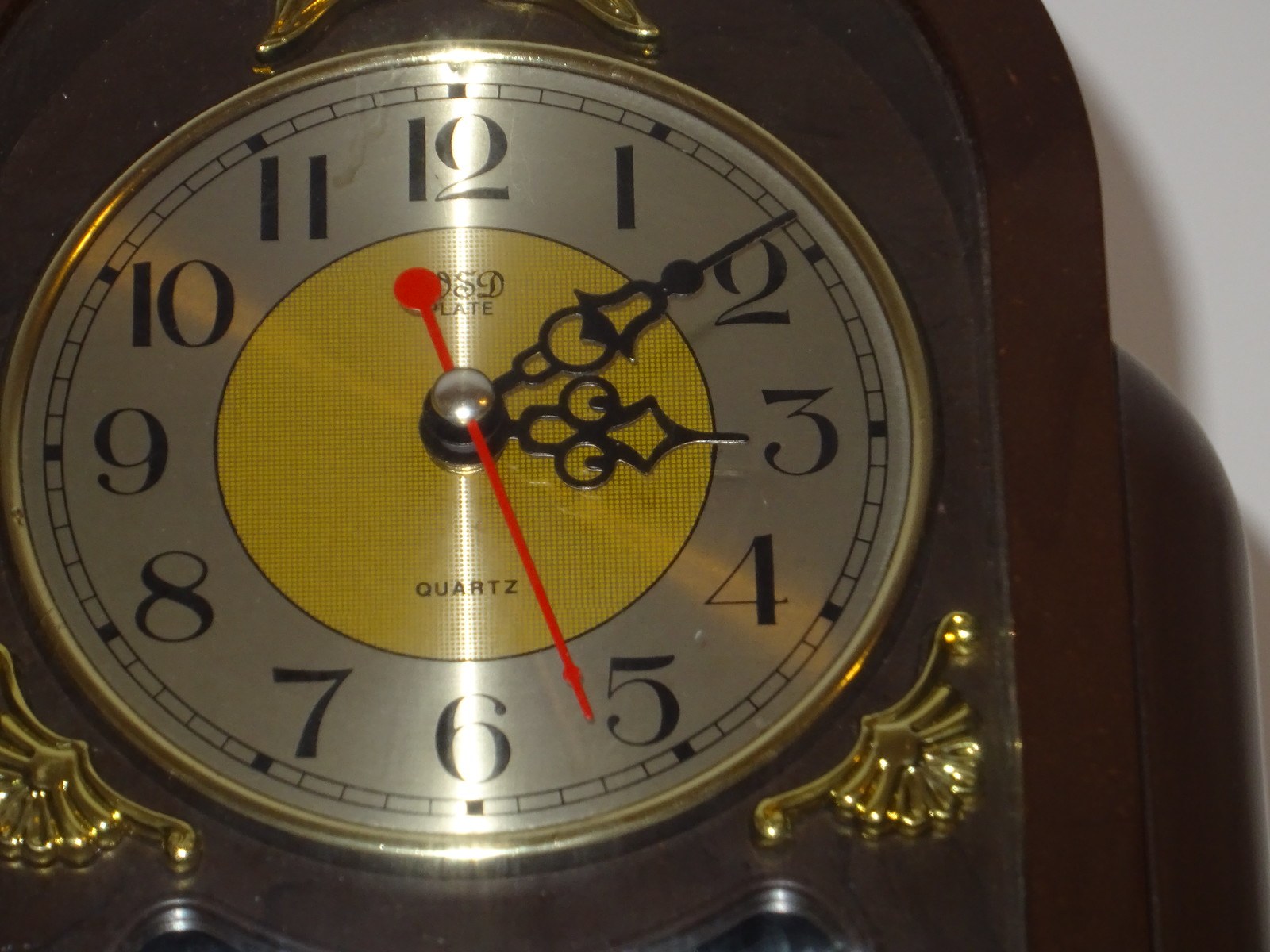This is a detailed close-up photograph of the face of an elegant freestanding wooden clock. The clock features a silver-colored base plate encircled by a gold ring. At the center of the clock face is a prominent yellow disc, adorned with ornate black minute and hour hands, and a long, thin red second hand. A partially obscured label, blocked by the minute hand, appears on the yellow disc, likely indicating "SD plate," and the word "quartz" is clearly printed in black letters below it. The clock numerals are Arabic, sequentially positioned from 1 through 12.

The frame of the clock is constructed from dark wood, featuring an inverted U-shape with gently curved lower shoulders. At the top of the clock face, a gold crest ornamentation with intricate spiraling curves adds a touch of opulence. Matching spiral crests are located on the left and right sides at the bottom of the clock face, providing symmetry and balance.

Light reflects off the clock face, suggesting the presence of a protective glass cover. The clock rests gracefully against a pristine white wall, amplifying its sophisticated and timeless design.